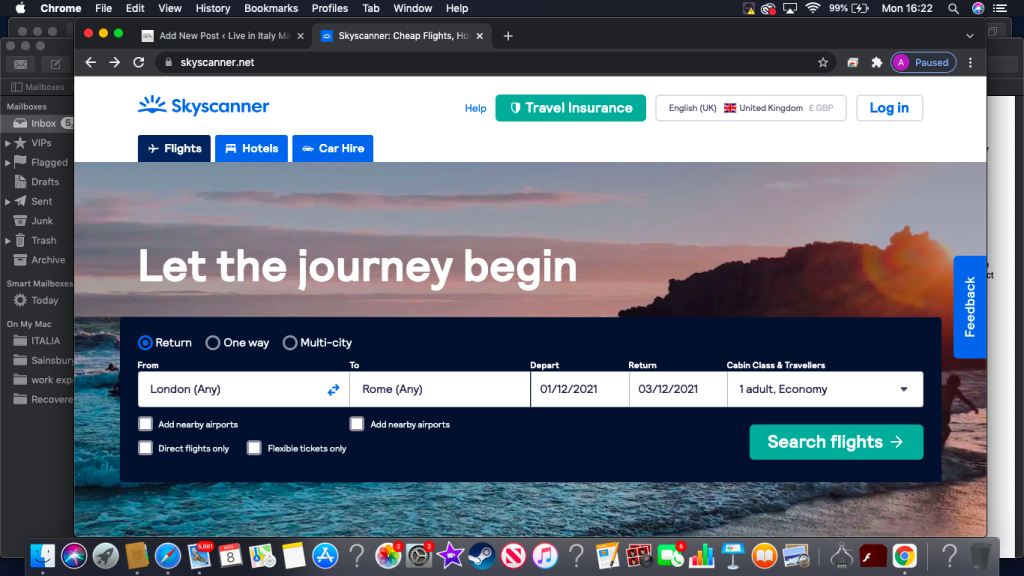Here's a cleaned-up and detailed caption:

---

This screenshot displays a Chrome browser window on a MacBook in dark mode, with the interface adorned in a dark charcoal color. At the top-left corner, an Apple icon is followed by white text listing the menu options: "Chrome," "File," "Edit," "View," "History," "Bookmarks," "Profiles," "Tab," "Window," and "Help." On the right side of the top bar, several small icons are visible, including Wi-Fi and battery indicators, along with the date and time set at 16:22 on a Monday. A magnifying glass icon is also present. 

Below the top bar, two Chrome tabs are open. The first tab is labeled "Add New Post - Live in Italy," and the second tab is labeled "Skyscanner - Cheap Flights." The second tab is the active one, displaying the Skyscanner homepage. At the top of the Skyscanner page, a white banner features a blue icon of a setting sun, accompanied by "Skyscanner" in blue font. To the right of the Skyscanner logo, "Help" is written in blue, followed by a gray rectangle with "Travel Insurance" in white text.